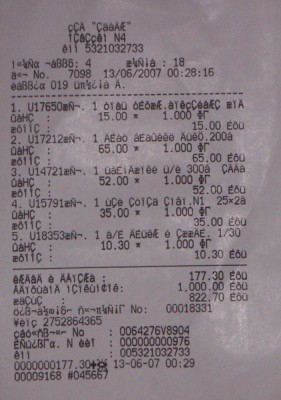A white, standard-looking receipt, written in a foreign language, making it difficult to decipher. At the top of the receipt, there's a date: 13-06-2007. The receipt lists five purchased items. The total amount at the bottom is 822.70. Comparing it to an American receipt, this figure appears to be the final total, although the specific items bought are unclear due to the language barrier.